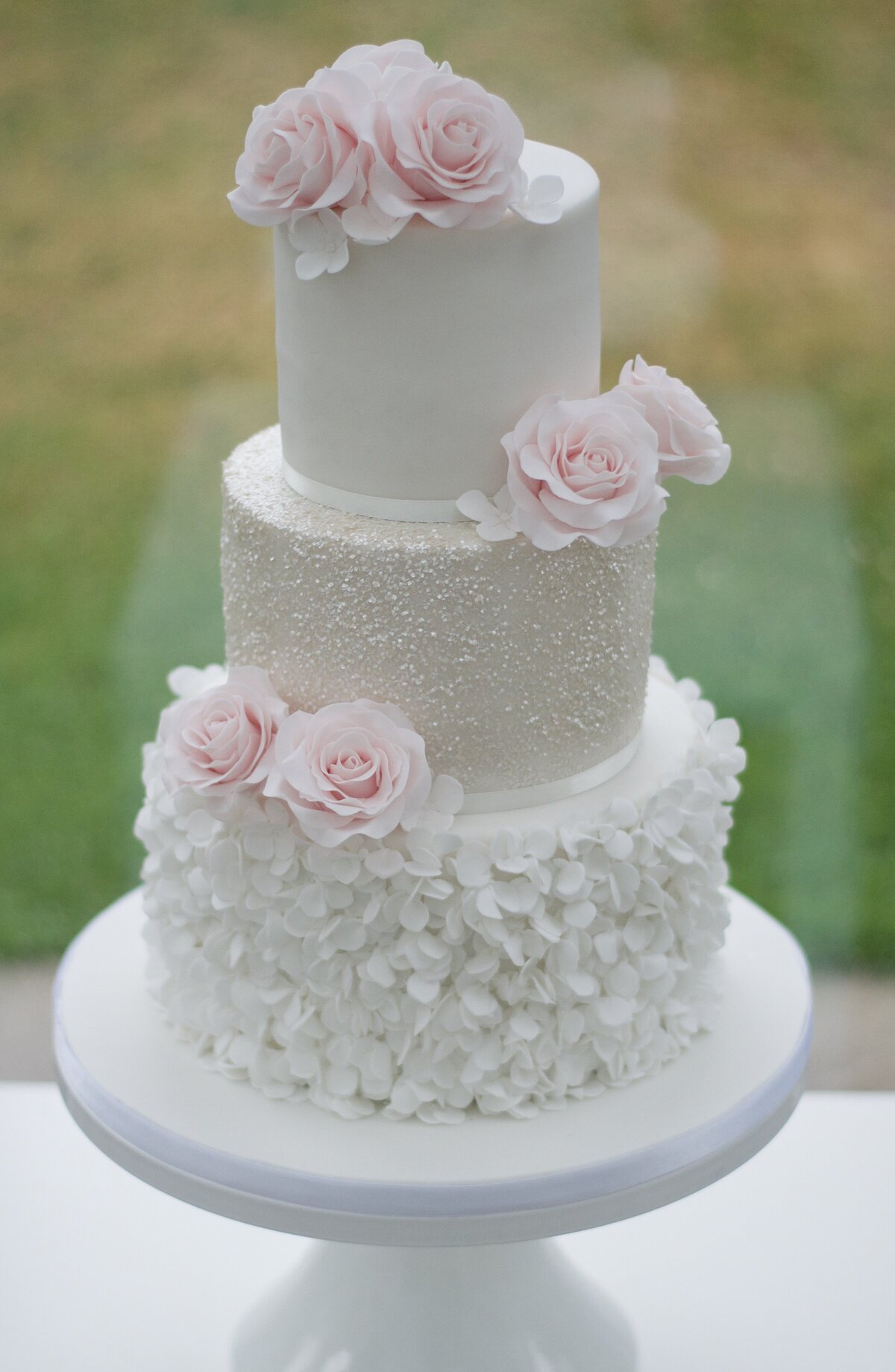This image features an elegant three-tier wedding cake displayed on a white ceramic pedestal cake stand. Each tier of the cake features distinctive decorations and a harmonious color scheme of white and the palest pinks. The bottom tier is lusciously adorned with delicate white petals giving it a textured floral appearance. Above it, the middle tier has an antique gold hue with a subtle popcorn bubbly texture, softened by evenly spaced, very light pink roses. The topmost tier is smooth and pure white, crowned with three light pink roses. In total, there are pairs of these roses on the bottom and middle tiers as well. The cake exudes a sophisticated and feminine aura, with the background exhibiting a blurry, muted green and yellow palette that suggests an outdoor setting. The overall presentation hints at a wedding cake, yet it's equally suitable for any elegant special occasion.